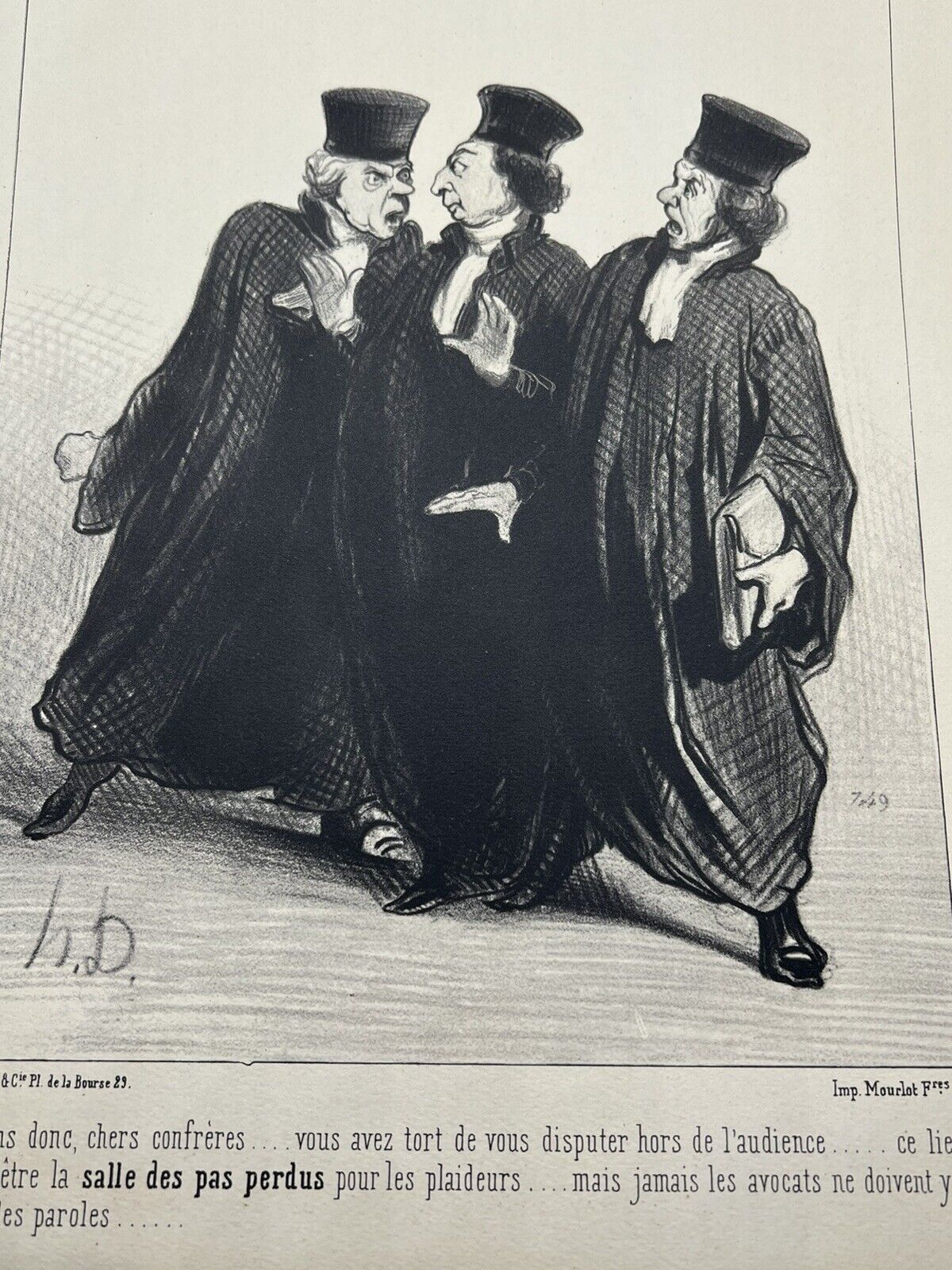This detailed description combines elements from all three original captions:

This black-and-white illustration appears to be taken from a very old newspaper, likely from the 18th or 19th century. It features three animated men who look like they could be judges or lawyers, each donning long black robes and tall hats that are flared at the top without brims. They also appear to be wearing wigs that extend from the back of their hats. The man in the middle has both hands extended upwards, seemingly trying to separate the other two men who are in an argument. The man on the left has his hand clenched in a fist and appears to be yelling at the man on the right, who looks surprised. There is a satchel being held by one of the men, adding to the sense of authority. The illustration is done in a detailed pencil style with extensive crosshatching. At the bottom, there's French text reading "Dans chers confrères, je vois toutes vos disputes hors de l'audience. La salle des postes produit pour les plâtres. Mieux jamais les avocats n'aient," indicative of a courtroom or legal context. Additionally, the abbreviations "HD" or "HB" and the numbers "seven of nine" or "seven four nine" appear near the artist’s signature in the lower left-hand corner. The style, attire, and language all suggest this scene is set in a European country, possibly France.